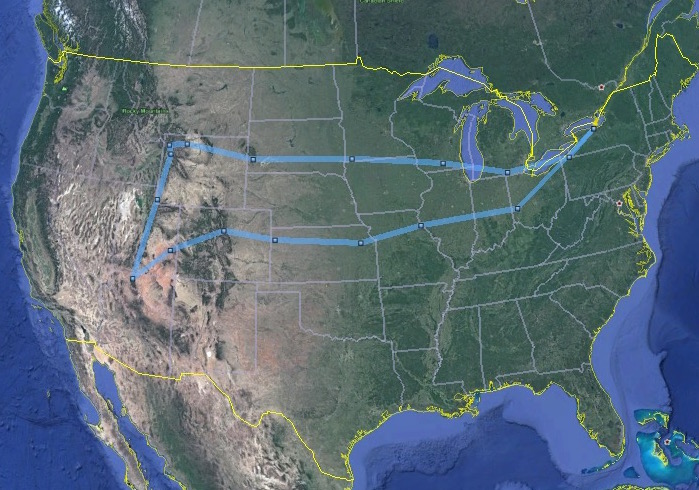The image depicts a detailed satellite view map of the United States, with parts of Canada and Mexico visible. The outline of the United States is highlighted with a thin yellow line, while the states within are outlined in white or light gray. A prominent, thick blue line marked by dots traverses from upstate New York, through Pennsylvania, and spreads laterally across the central United States, passing through regions like Utah, Colorado, Kansas, and Missouri. It loops back through areas such as Chicago and Detroit, eventually returning to its starting point in upstate New York. The map features color-coded topographical details, with green regions indicating plains, and brown areas representing mountainous terrains. The oceans surrounding the landmasses are depicted in shades of blue and purple, and the map also shows various islands in the Caribbean. This appears to be a travel-oriented map, possibly akin to Google Maps, but does not include insets for Hawaii or Alaska.